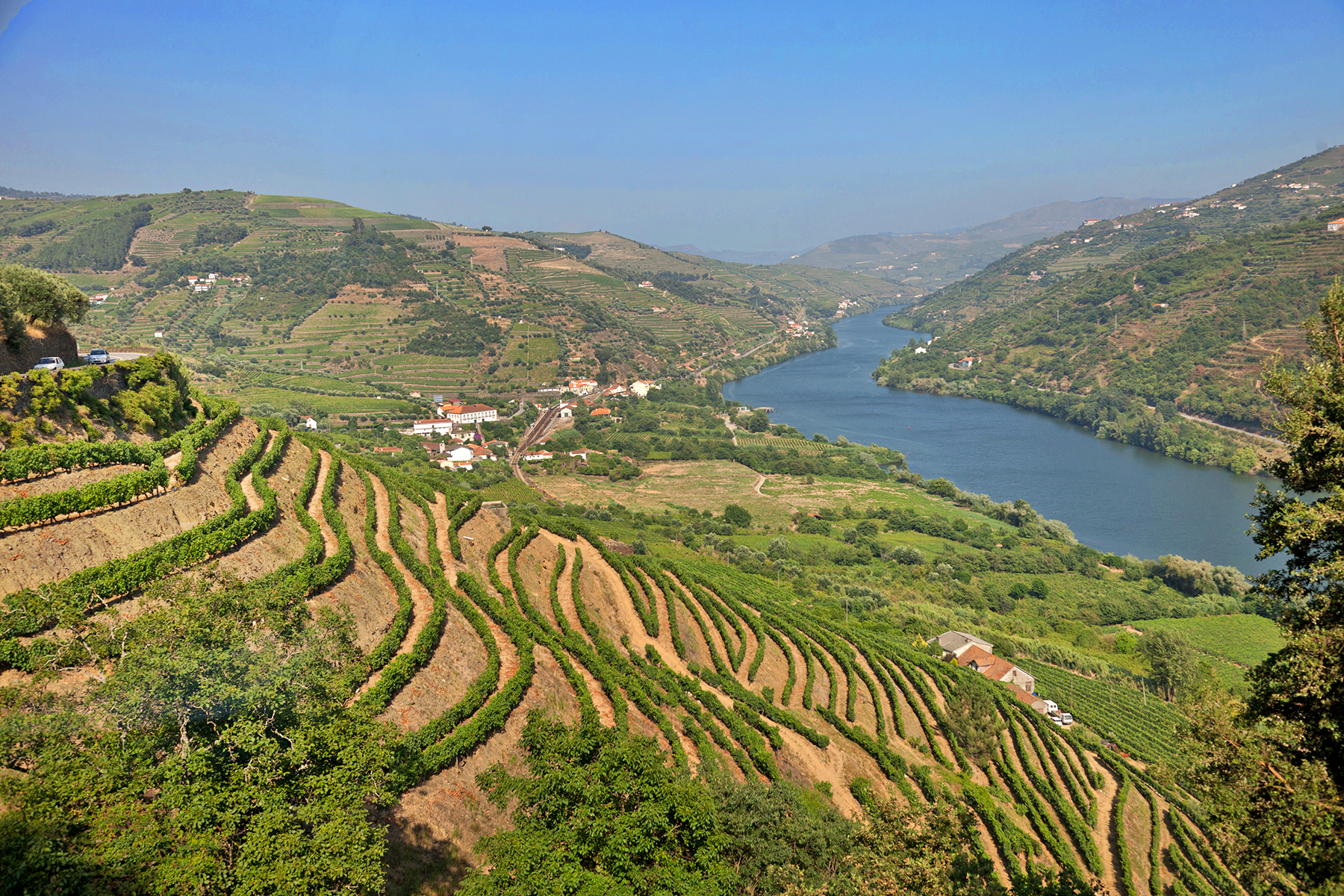This image depicts a picturesque countryside scene, characterized by rolling hills that dominate the landscape and extend into the background. The vibrant color palette includes an expansive clear blue sky with a slight haze, lush green and brown hillsides, and scattered patches of white, red, and orange from various elements within the photo.

In the center of the image, a calm, narrow river meanders through the hilly terrain, flanked by landmasses with considerable elevation changes. On the left side of the image, several homes and small communities are nestled among the hills, some of which seem to feature commercial developments. The hillside closest to the camera in the foreground showcases sculpted shrubs arranged in decorative wavy lines, indicating human cultivation and design.

The right side of the photo mirrors the left but with fewer houses dotting the landscape. The overall setting suggests a rural, mountainous countryside with a harmonious blend of natural beauty and human habitation. The photo captures the serene coexistence of the rugged terrain, clear skies, tranquil water, and the curated greenery on the cultivated hillside.